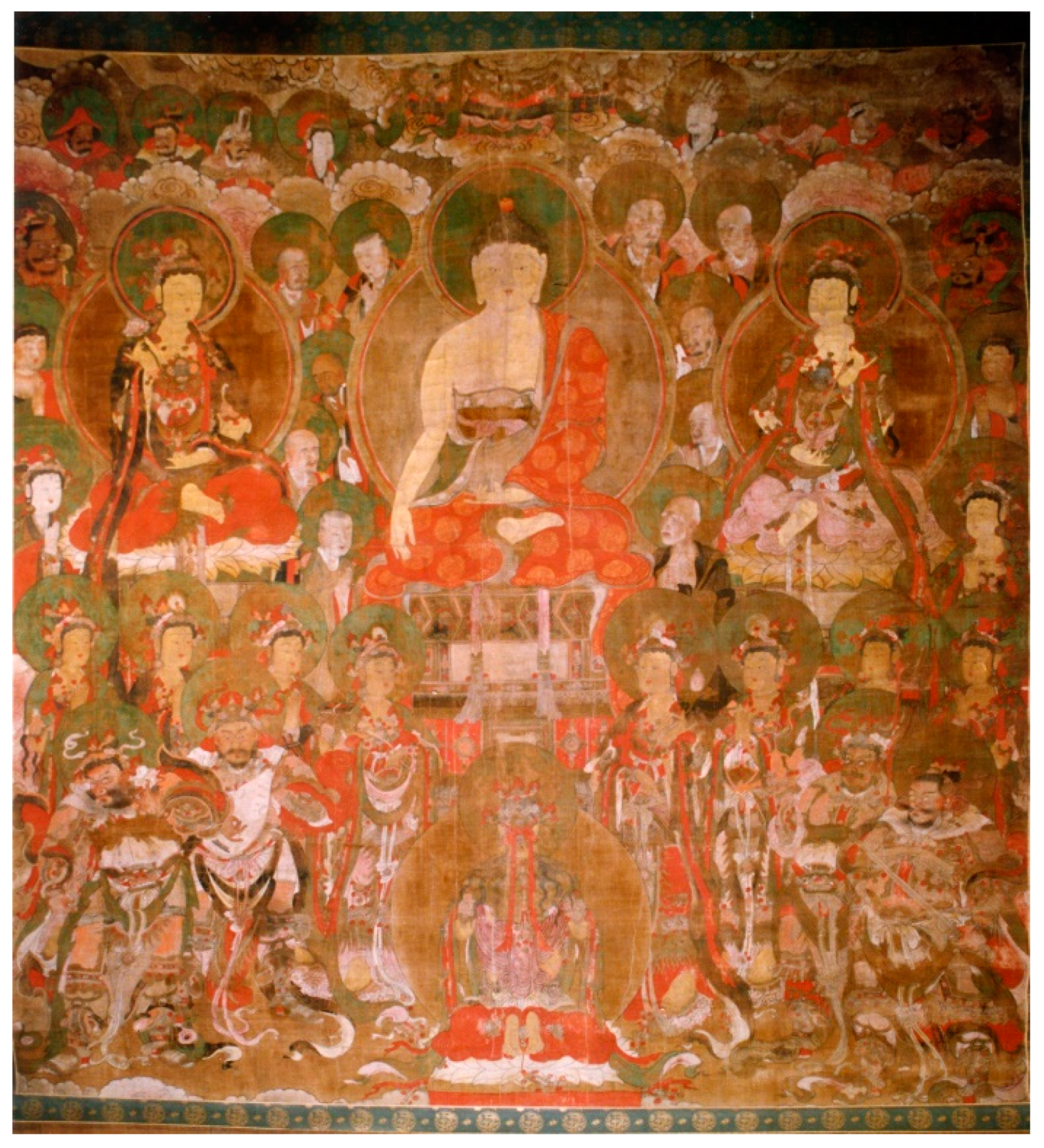This photograph captures a large, ancient tapestry with a distinctly Asian, likely Chinese, aesthetic. The tapestry is bordered by intricate patterns featuring green ovals and yellow circles, which frame the central scene. In the middle, three figures serve as the focal point: a man adorned in vibrant red, flanked by two women—one dressed predominantly in red and the other in pink. These figures are seated cross-legged, evoking a sense of religious or historical significance. Surrounding them, approximately fifty characters populate the tapestry, many of whom are women, though some men with beards and distinct attire can be seen toward the bottom. The overall tapestry displays a faded, yet still vibrant color palette dominated by reds and greens, with characters adorned in ornate, almost samurai-like garb. This piece appears to be a photograph of an aged fresco or painting, possibly housed in an ancient building, hallway, or museum, capturing the essence of a rich cultural and artistic heritage.